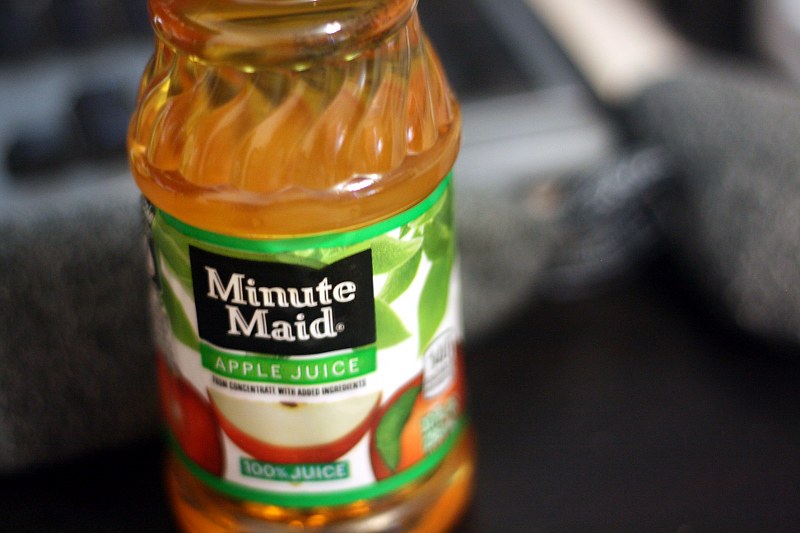This detailed photograph features a single-serve bottle of Minute Maid apple juice as its focal point. The bottle is clear plastic, filled with the light golden color of apple juice. Though the lid is not visible, the top part of the bottle and the juice within can be clearly seen. The label, wrapped around the bottle just below the neck, displays the brand "Minute Maid" in white letters on a black background. Beneath this, the words "apple juice" are prominently displayed in white text against a green background. The label also features an image of fresh-cut apple slices and green leaves, suggesting a natural and healthy beverage. Additionally, the label indicates that the juice is 100% pure. The background of the photograph is intentionally blurred, giving an indistinct glimpse of potential shapes and possibly hinting at a kitchen or desk setting, but without enough detail to be certain. This inviting and delicious presentation emphasizes the drink's purity and natural appeal.